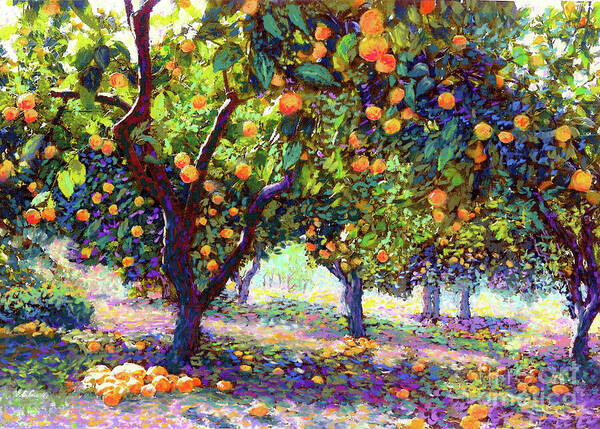The hand-drawn painting depicts a vibrant orchard, potentially of oranges or tangerines. Dominating the left side is a prominently detailed tree with a thick trunk and branching limbs adorned with abundant leaves and hanging oranges. The landscape is alive with multiple similar trees stretching into the background on the right, each laden with the same vibrant fruit. The ground is scattered with fallen oranges, some amassed into a conspicuous pile on the left, and interspersed with grass and possibly flowers. Distinctly, some tree trunks and shadows are painted in a striking purple hue, contrasting with the lush green foliage. A path weaves through the center behind the main tree, leading to a bush on the left. The trees exhibit a gnarly structure, with twisted branches and trunks adding to the rustic charm. A semi-transparent watermark in the bottom right corner, partially legible, prominently featuring the word "art," signifies the creator's mark.